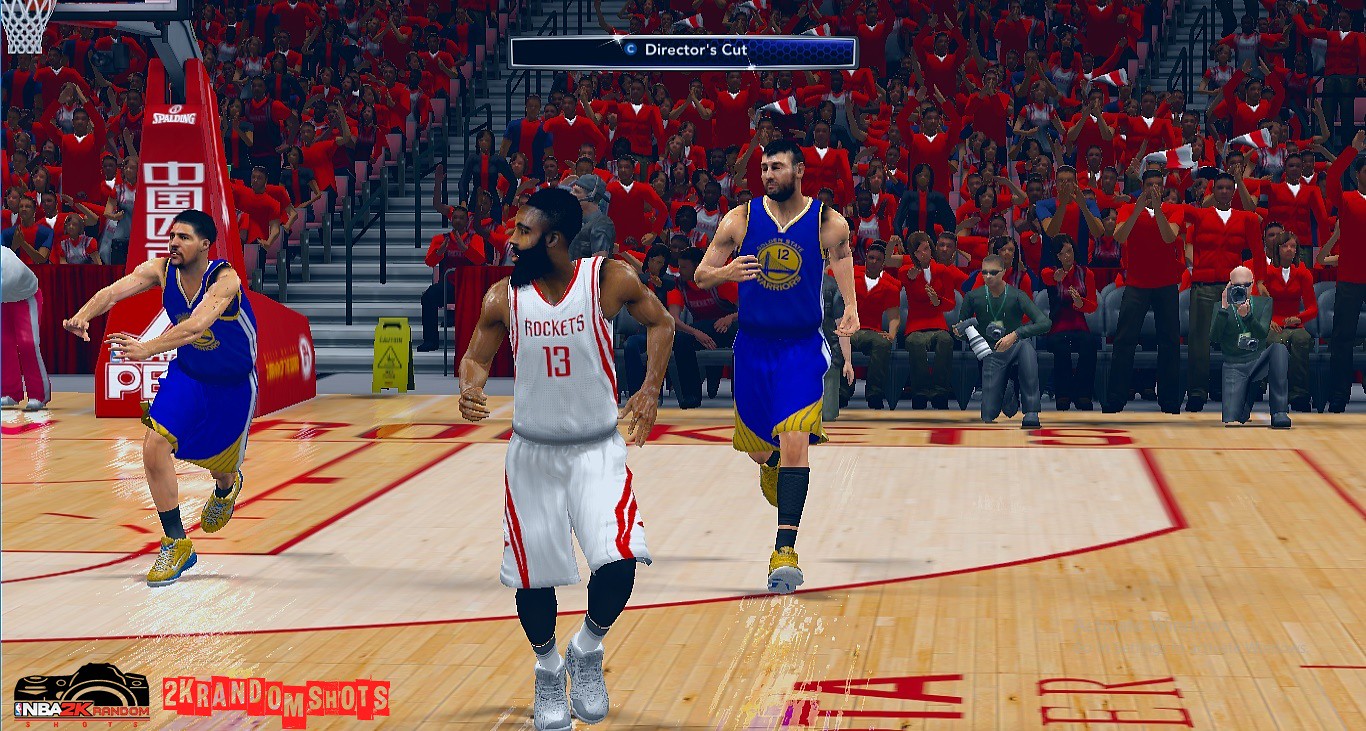The image is a detailed screenshot from what appears to be a basketball video game. The game is set in a realistic stadium filled with numerous spectators, most of whom are dressed in red shirts. The center of focus is on three basketball players on a well-defined wooden basketball court marked with red and white lines. The player in the middle wears a white uniform emblazoned with "ROCKETS" in red and the number 13, while the players on either side sport blue and yellow uniforms, with the player on the right wearing number 12. Above the court, a rectangular gradient blue banner displays the words "Director's Cut." At the bottom left corner of the image, the text "NBA2K Random Shots" is prominently featured with a red backing and white font. Additionally, a caution sign can be seen near the hoop, indicative of detailed environmental elements in the game's design. The hoop itself is branded with Asian characters. Spectators, photographers in green tops, and other dynamic elements of the crowd enhance the immersive atmosphere of the scene, capturing the energy and realism of an NBA game.